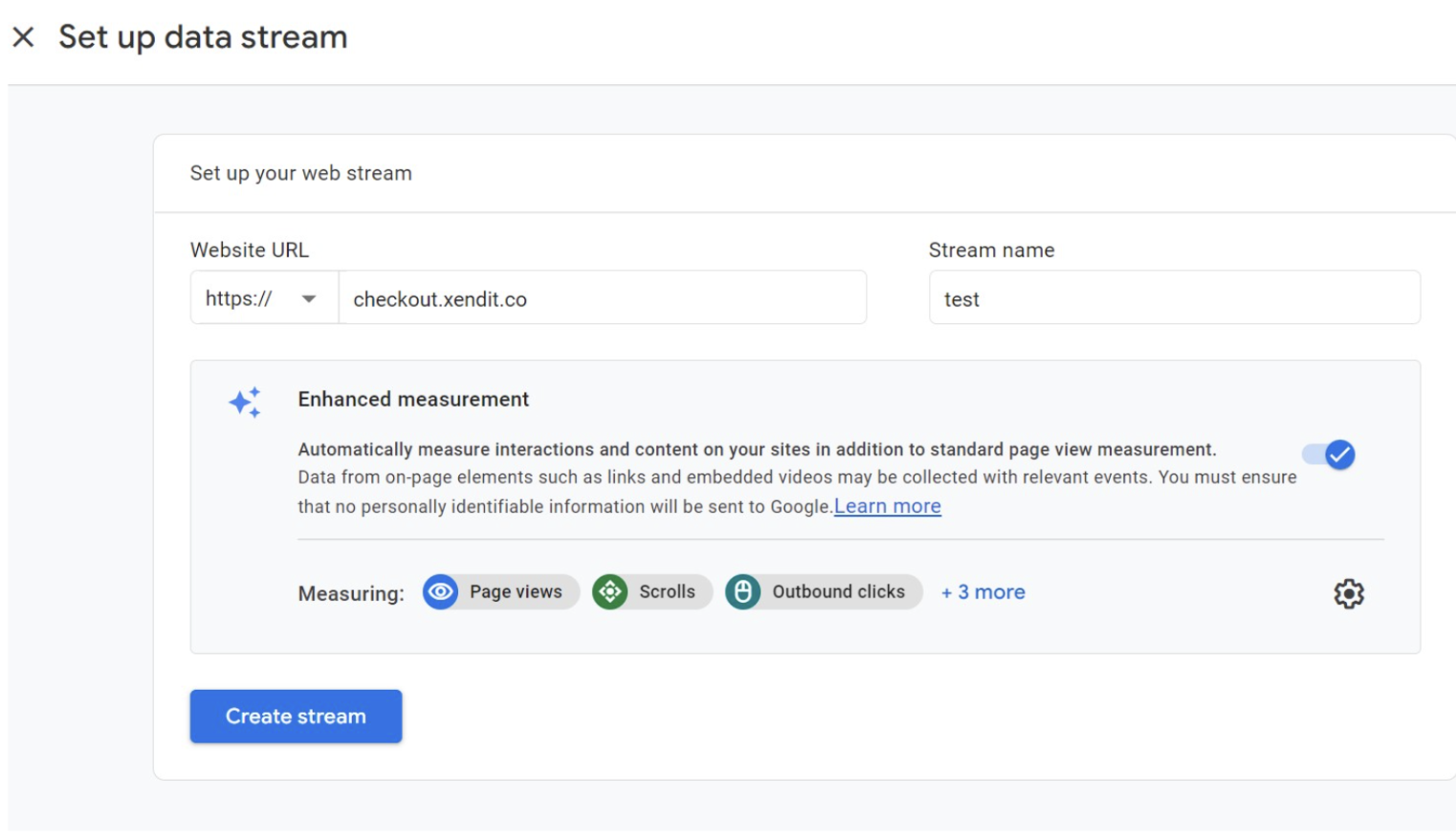The image features a rectangular setup interface for establishing a web data stream. At the very top of the interface, there is an "X" icon. Immediately below that, the header "Set Up Data Stream" is displayed. The top section of the rectangle is white, transitioning to a light gray color as the background for the main content.

The primary content area is a white rectangular box with the instruction "Set up your web stream" at the top. Beneath this, there's a line followed by the label "Website URL" accompanied by a dropdown menu prefilled with "https://". Adjacent to this dropdown is a data field containing the URL "checkout.xendit.co."

Below this URL field, the label "Stream Name" appears, also including a data field that contains the prefilled text "test."

Further down, there is a gray rectangular box with the text "Enhanced measurement automatically measures interactions and content on your sites in addition to standard page views. Measurement data from on-page elements such as links and embedded videos may be collected with relevant events. You must ensure that no personally identifiable information will be sent to Google. Learn More." 

On the left side of this gray box, there is a blue toggle switch, indicating that the enhanced measurement feature is activated. Below the toggle, the text outlines the types of data being measured: "page views, scrolls, outbound clicks plus three more."